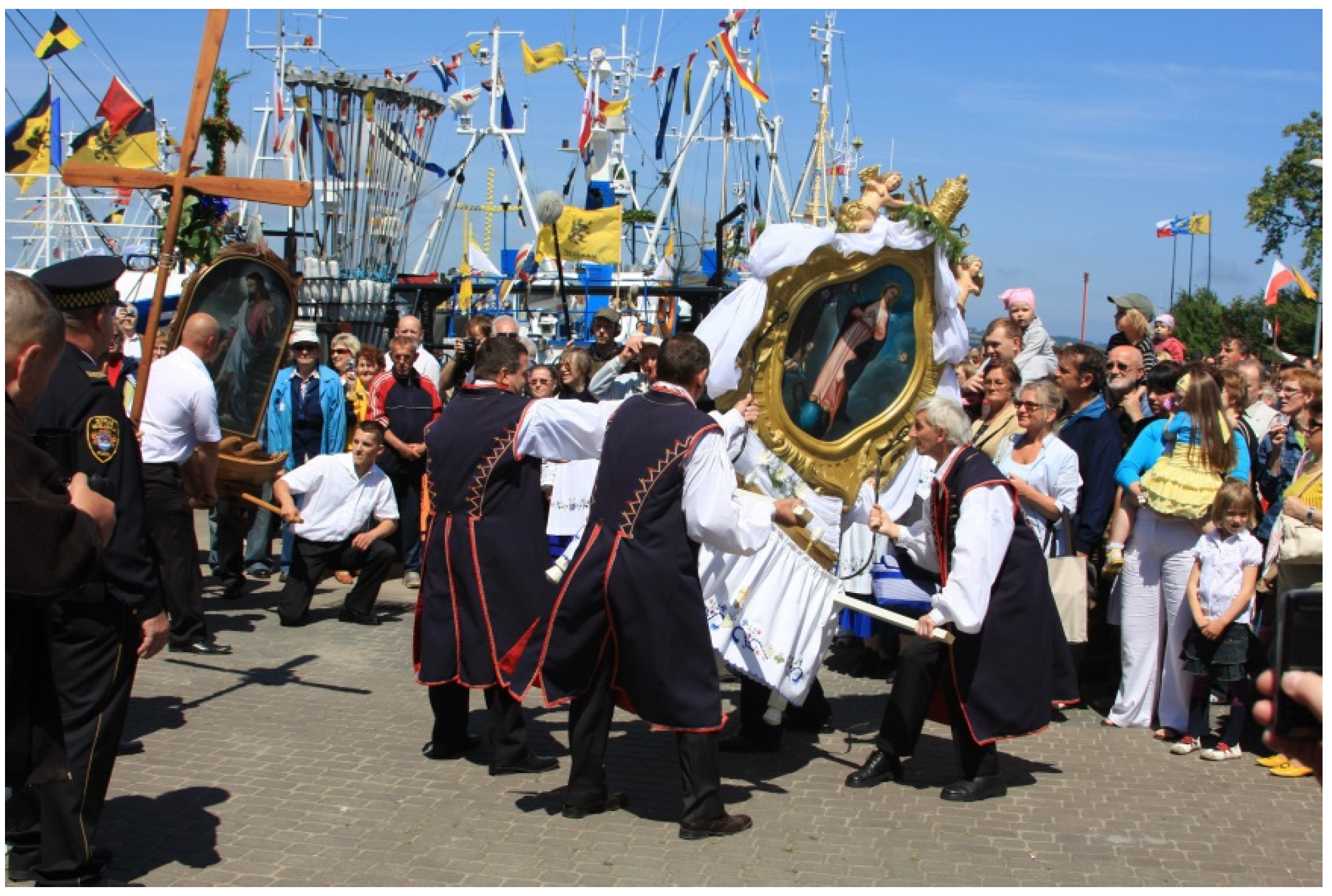In this photograph of what appears to be a lively historical reenactment festival held on a beautiful sunny day with clear blue skies, we see a group of participants dressed in elaborate pirate or Renaissance garb. The central figures are adorned in long, black or charcoal gray outfits with ornate red trim and white billowy shirts underneath. They carry a gilded, white-clothed structure—a golden treasure-like piece adorned with intricate decorations and a painting of a lady on it—on wooden poles, giving the impression of a ceremonial or religious artifact.

The crowd around them is a mix of everyday spectators, dressed in typical summer attire with many wearing sunglasses, adding to the vibrant, contemporary atmosphere. In the backdrop, an impressive pirate ship or naval vessel is docked on the water, decorated with various colorful flags—yellow, black, red, and blue—making it a striking and colorful sight. To the left side of the image, a uniformed police officer, dressed in either dark blue or black, supervises the event, ensuring the crowd's safety. The scene takes place on a gray brick roadway or sidewalk, adding to the historical ambiance of this unique festival.